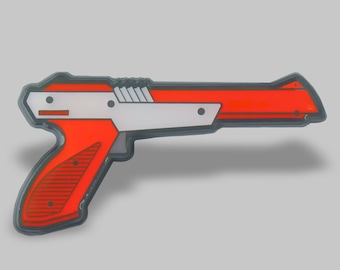The image showcases a realistic portrayal of a toy gun, set against a pristine white background. The sole object in the image casts a subtle gray shadow below and slightly behind it, adding depth. The toy itself is designed to resemble a classic Nintendo light gun, famous for its use in games like Duck Hunt.

The gun is framed within a flat, gun-shaped piece of material, which features a gray border running around its entire silhouette. The gun's body is primarily a vibrant red, complemented by a gray section above the trigger area. This section includes darker gray accents that contribute to the overall vintage design. The trigger of the gun is distinctly dark gray, emphasizing its functionality. The meticulous color scheme and design details evoke a sense of nostalgia for the iconic Nintendo gaming accessories.